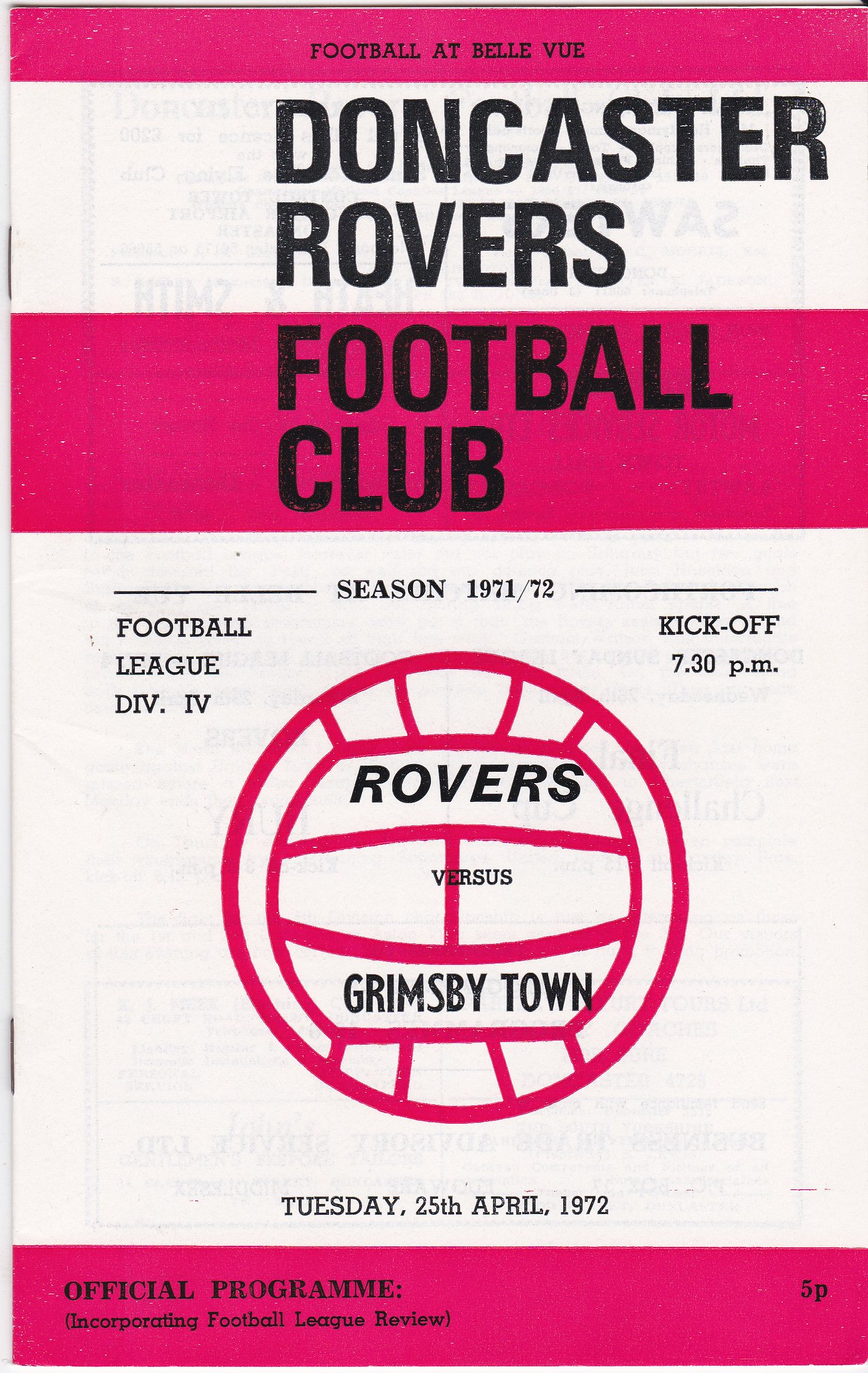The photograph depicts the cover of a vintage football program for a match at Bellevue between Doncaster Rovers and Grimsby Town. At the top of the program, a dark pink stripe bears the title "Football at Bellevue" in black letters. Below this, on a white background, "Doncaster Rovers" is prominently displayed in black capital letters. Further down, another pink stripe contains the text "Football Club" in black. Centrally placed on the cover is a hand-drawn soccer ball with red stripes. In the middle of this ball, the text "Rovers versus Grimsby Town" is clearly printed. Above the ball, small black letters indicate the season "1971-72," with "Football League Division Four" on the upper left side and the kickoff time "7:30 p.m." on the upper right. Beneath the ball, the date "Tuesday, 25th April, 1972" is printed. At the very bottom, another pink stripe features the words "Official Program" in black, along with "5p" (five pence) indicating its price, and the phrase "Incorporating Football League Review" in smaller print.